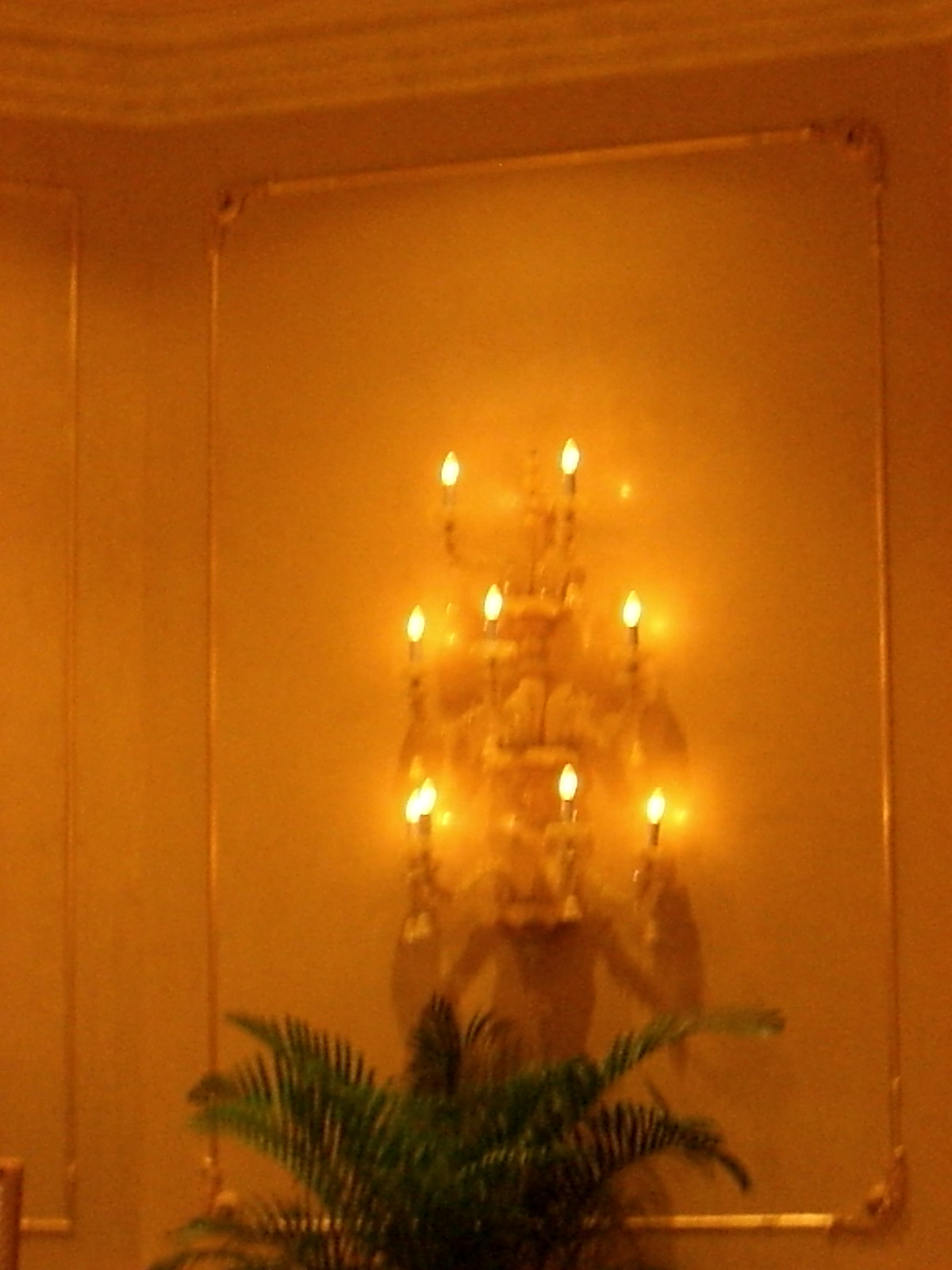This is a photograph of a grand, ornate decorative wall in what appears to be a fancy hotel with very high ceilings. The wall is adorned with intricate crown molding at the top and a large, ornate framed section in the middle, featuring a peach-colored wallpaper. Within this framed area, there is a complex, wall-mounted light fixture that resembles a chandelier. This elaborate light fitting consists of three tiers. The top tier has two electric candle-like bulbs, the middle tier has three, and the bottom tier has four. Each tier features arms extending outward, holding the candle-shaped bulbs that cast unique shadows resembling bodies and hands holding candles. Positioned below the light fixture is a lush, large fern plant with long stems and leaves sprouting outward. The overall setting exudes an air of opulence and elegance, typical of high-end hotel decor.